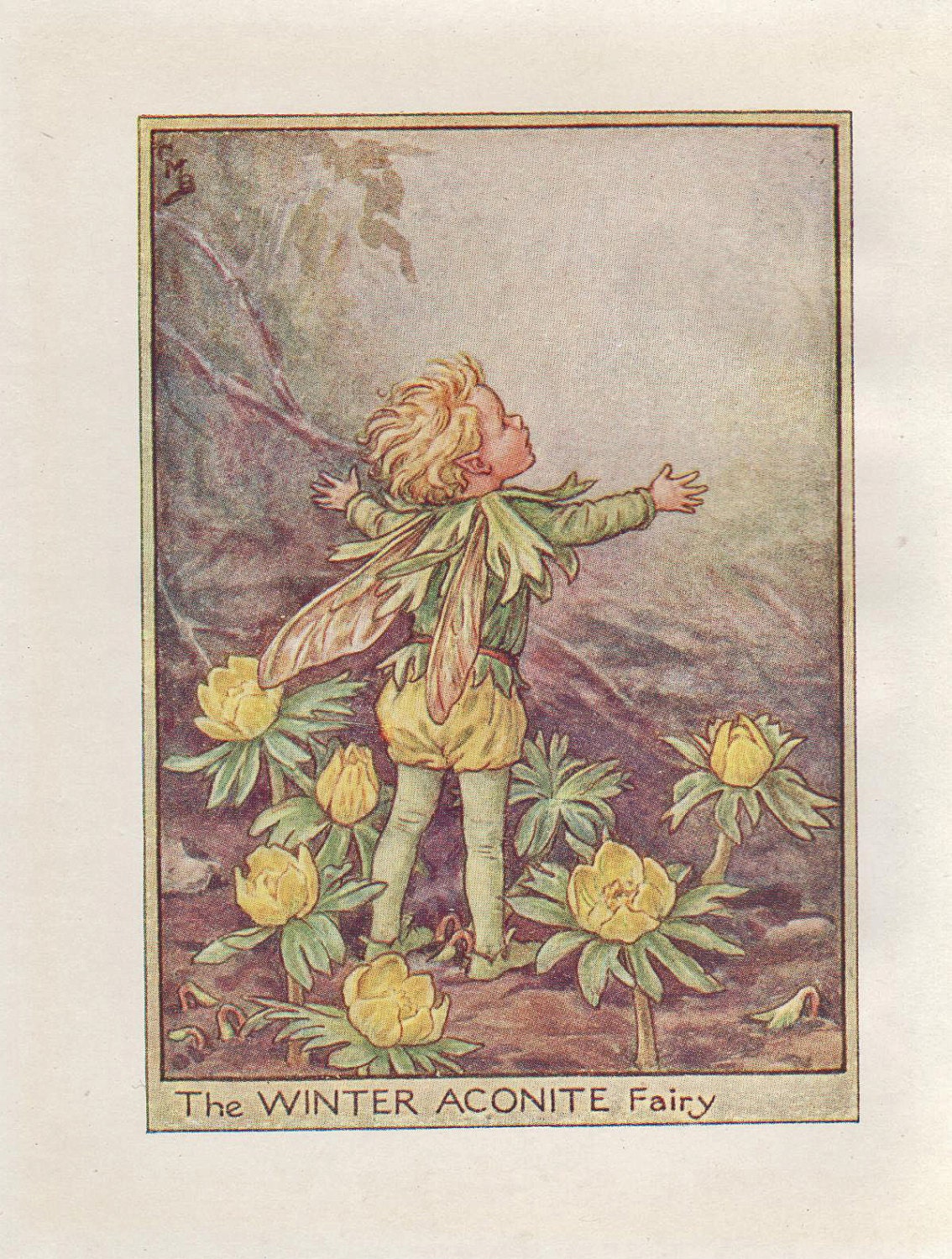In the image titled "The Winter Aconite Fairy," a charming illustration depicts a child-like fairy figure with wings and pointed ears, appearing to be a young boy with short, curly blonde hair. Positioned centrally, the fairy is shown in profile, facing slightly away but with his right side visible. He has his arms outstretched and seems to be looking upwards. The fairy is dressed in a whimsical outfit resembling elements of the forest: a green shirt with a leafy neckpiece, yellow bloomers, green tights, and pointy elf shoes. His silvery, translucent wings glisten, adding a magical touch to his appearance. The background features lush vegetation and trees, complementing the scene with a natural woodland ambiance. Bright yellow flowers, possibly crocuses or poppy-shaped blooms, surround the fairy, harmonizing with his yellow shorts. The image, which might be on a postcard or greeting card with a beige-grey cover and a greenish border, includes the title "The Winter Aconite Fairy" at the bottom, hinting at the fairy's connection to the enchanting winter aconite flowers. The ground is depicted with brown dirt, adding to the earthy and serene setting.